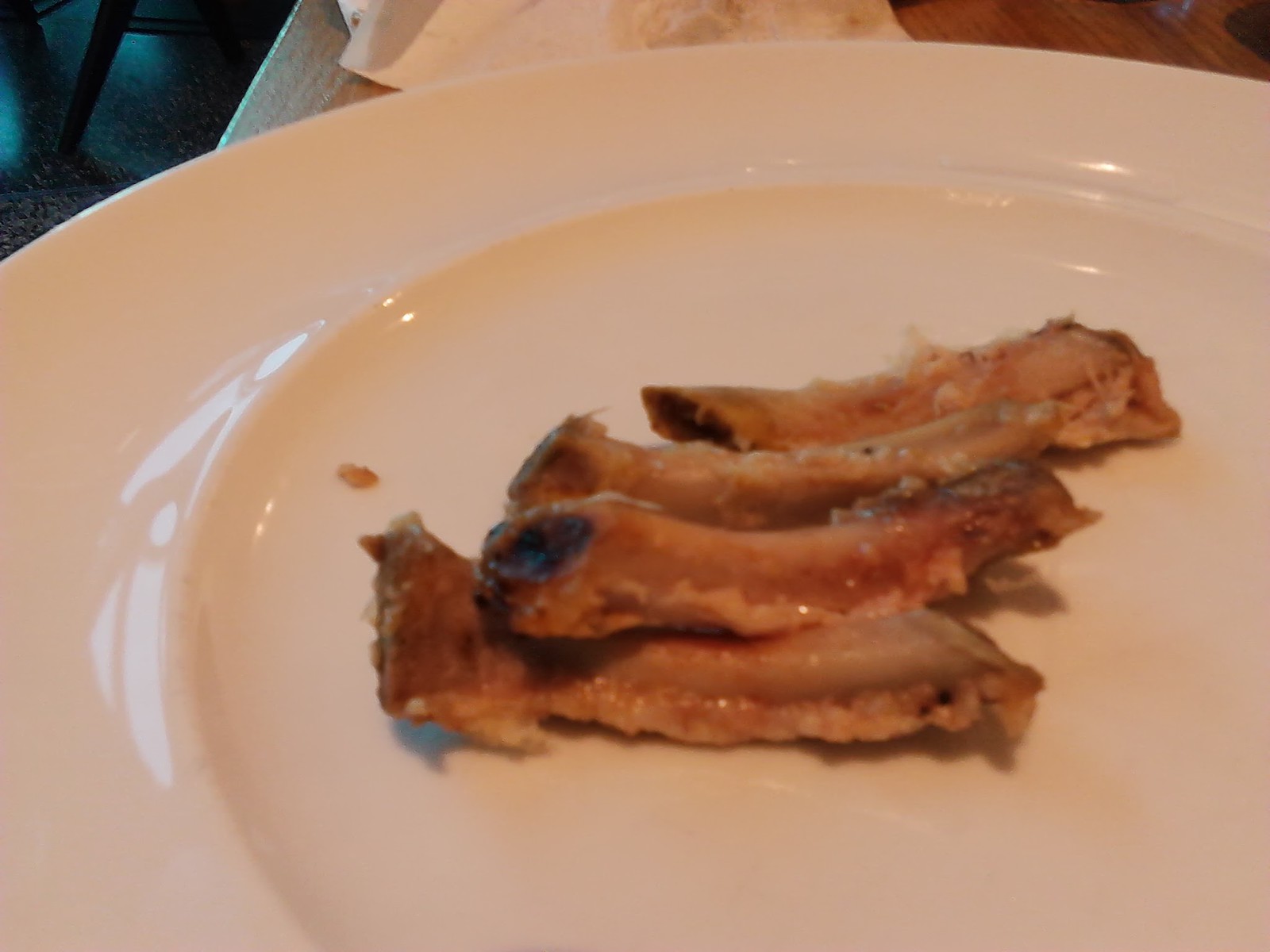The photograph captures a slightly blurry, close-up of a simple, white ceramic plate holding four well-eaten rib bones arranged vertically in a row. The bones, still bearing traces of meat and a reddish-orange, possibly barbecue, sauce, dominate the otherwise clean plate. In the background, on what appears to be a round wooden table, lies a greasy, white napkin with a portion of a chair and the floor also visible. Despite the poor lighting and out-of-focus elements, the image clearly conveys the remnants of a savory, home-cooked meal.